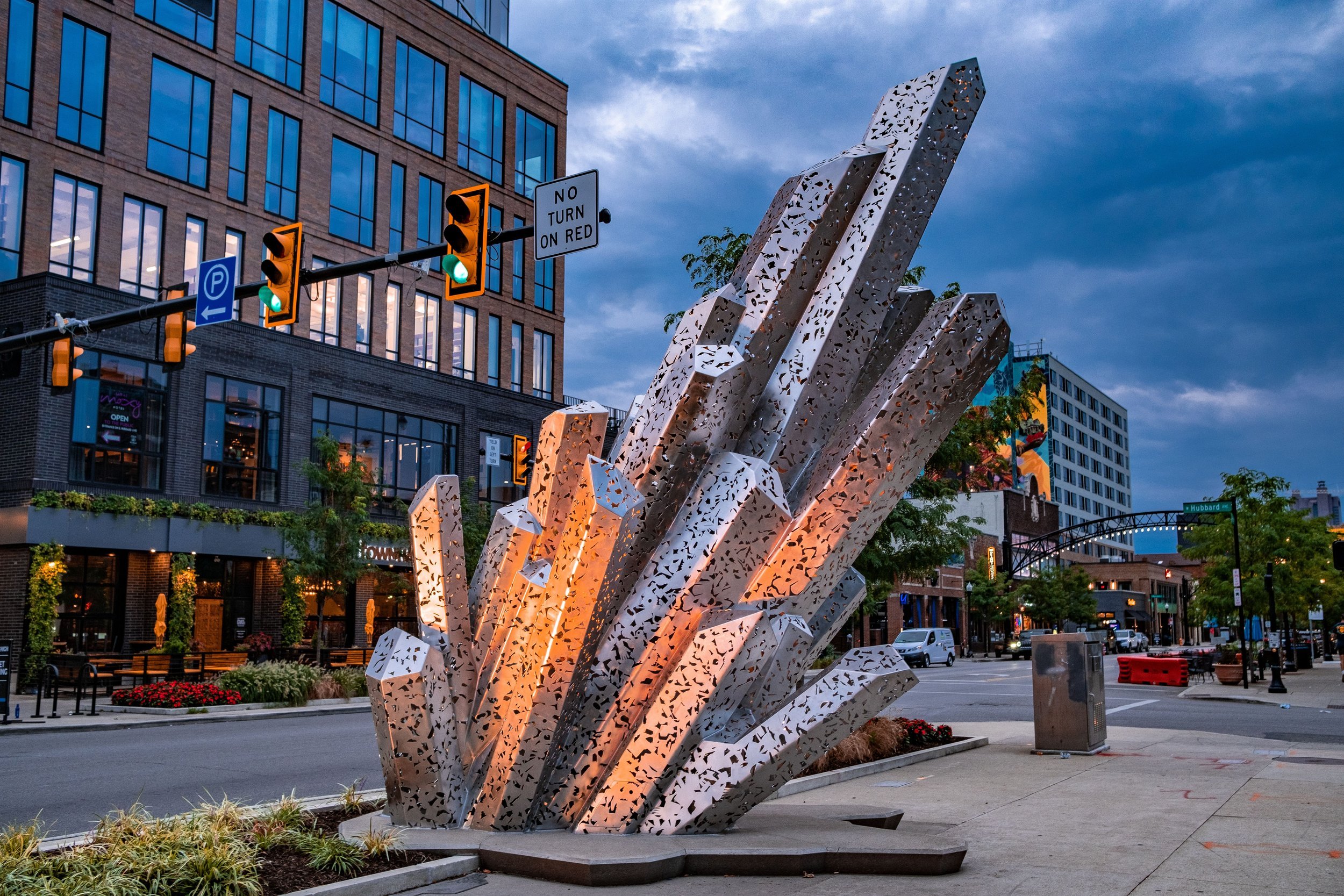This outdoor art installation features a striking, geometric sculpture resembling a cluster of large, reflective silver rectangular spikes with black speckles. Positioned at an angle, the sculpture's form evokes the image of a gigantic crystal emerging from the sidewalk. Surrounding the installation, there's a scene of urban life with a mix of residential and commercial buildings, some reaching up to six or seven stories high. A busy street with visible traffic, including a distant white van, and multiple green traffic lights define the vicinity. Signage such as a "No Turn on Red" and a parking sign with a blue "P" are noticeable. The setting includes a garden inset into the concrete pavement and permanent fixtures like a garbage can. The photograph captures a cloudy, overcast day with dark clouds above, reflecting the subdued lighting of the late afternoon or early evening. The overall composition blends elements of city infrastructure with the intriguing, modern aesthetic of public art.